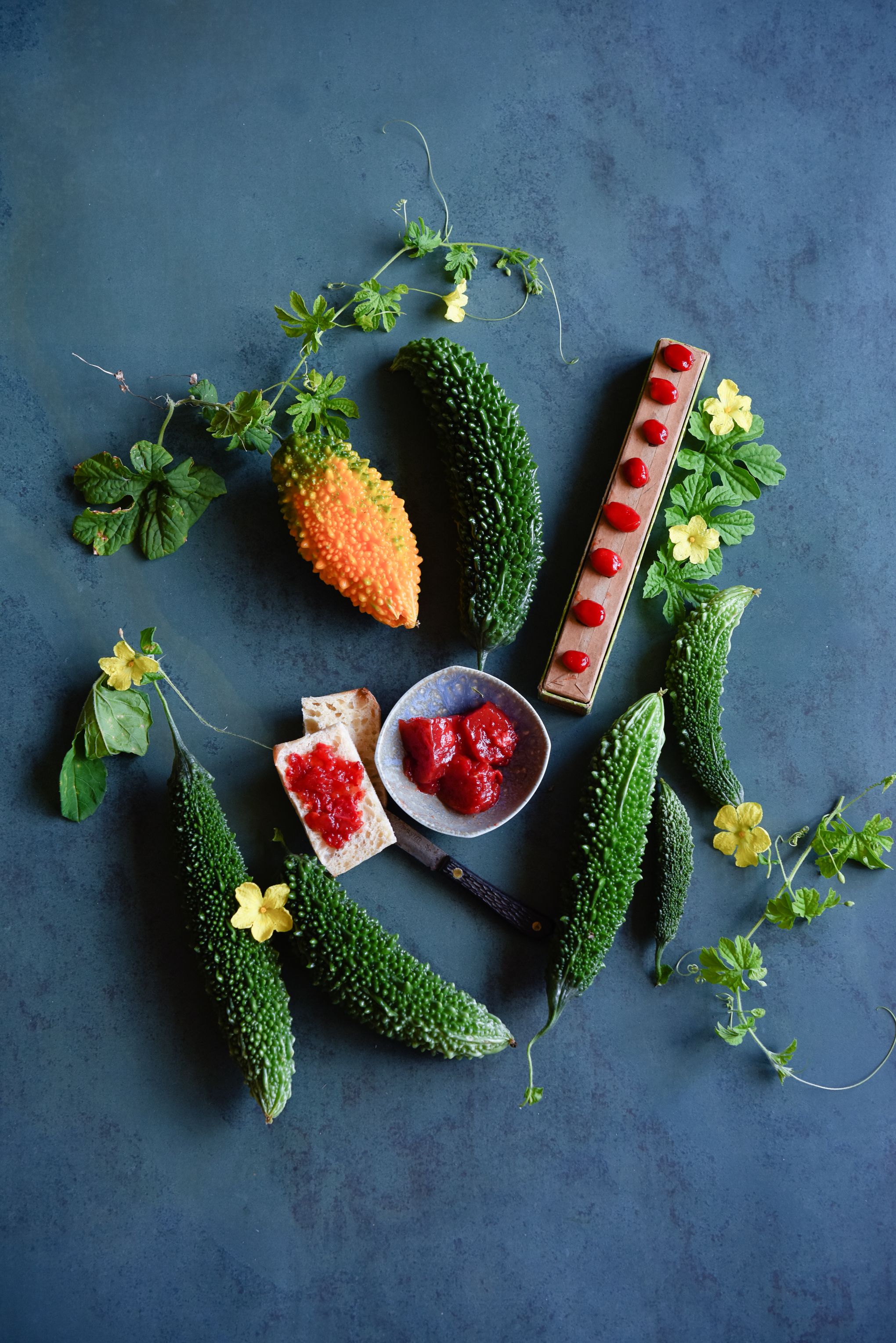The photograph showcases a variety of vegetables and food items laid out meticulously on a slightly rough-textured blue surface, likely a countertop or table. Central to the image are five to six bitter gourds, identifiable by their dark green, bumpy skins, with one distinct orange gourd among them. Each gourd remains attached to a green vine adorned with five-petaled yellow flowers. A small bowl containing red sauce or jelly is placed at the center of the layout. Adjacent to this bowl on the left are two rectangular-shaped crackers or biscuits, one of which has jelly spread on top, and a black-handled knife positioned beneath them. On the right side of the image, a narrow rectangular plate is artfully dotted with small droplets of sauce. The entire scene captures an intricate and somewhat exotic display, emphasizing the natural textures and vibrant colors of the vegetables against the muted backdrop.